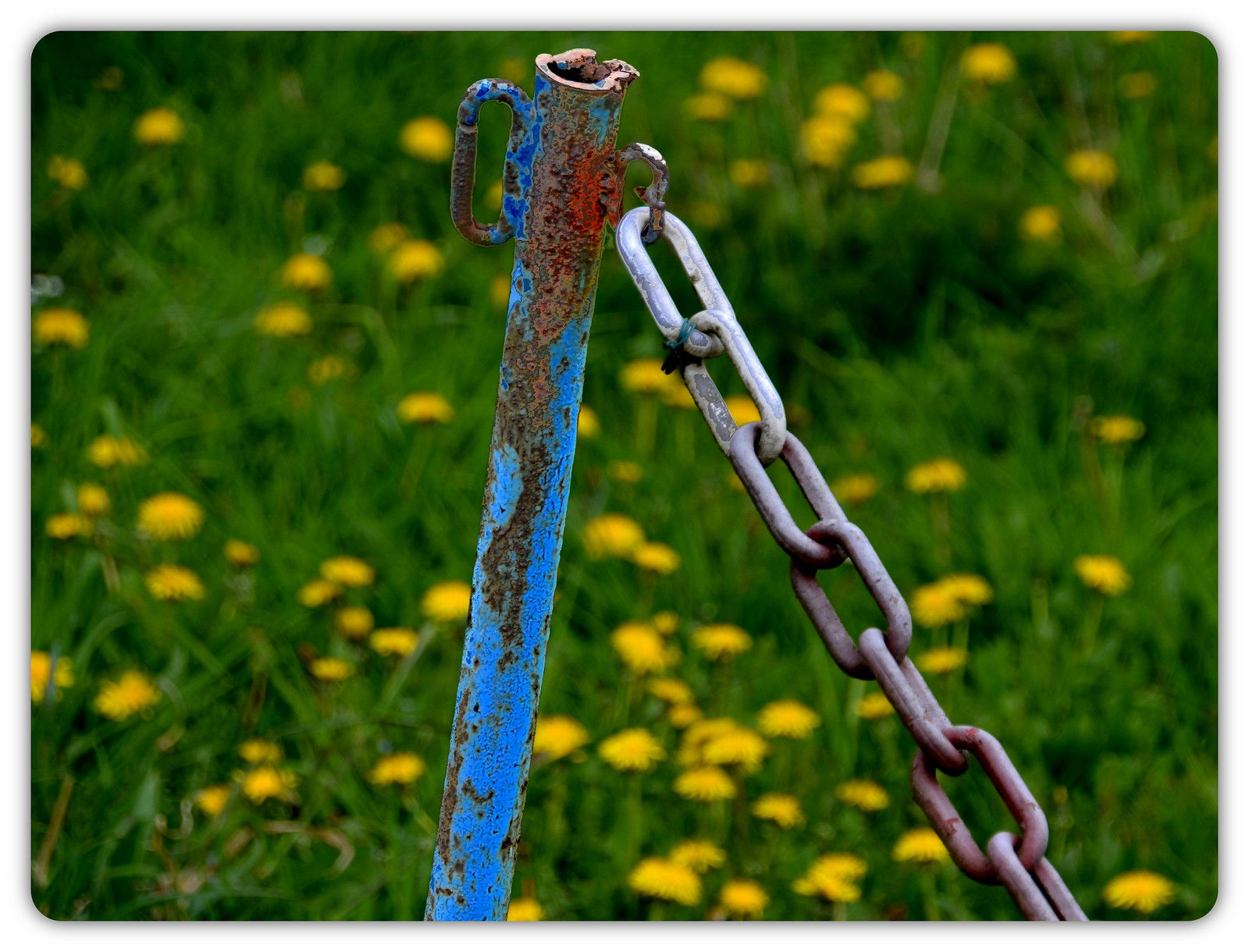The photograph features a weathered blue metal post jammed into the ground, with sections of red rust showing through the paint. Attached to the post is a silver metal chain, which is rusted at the bottom but has newer, shiny links near the top. Surrounding the post and chain is a lush, unmown field of thick green grass, scattered with numerous yellow dandelions and small wildflowers. The dampness of the setting is noticeable, suggesting it had recently rained or that the area is generally moist. The overall scene captures a simple, yet detailed rustic outdoor setting.